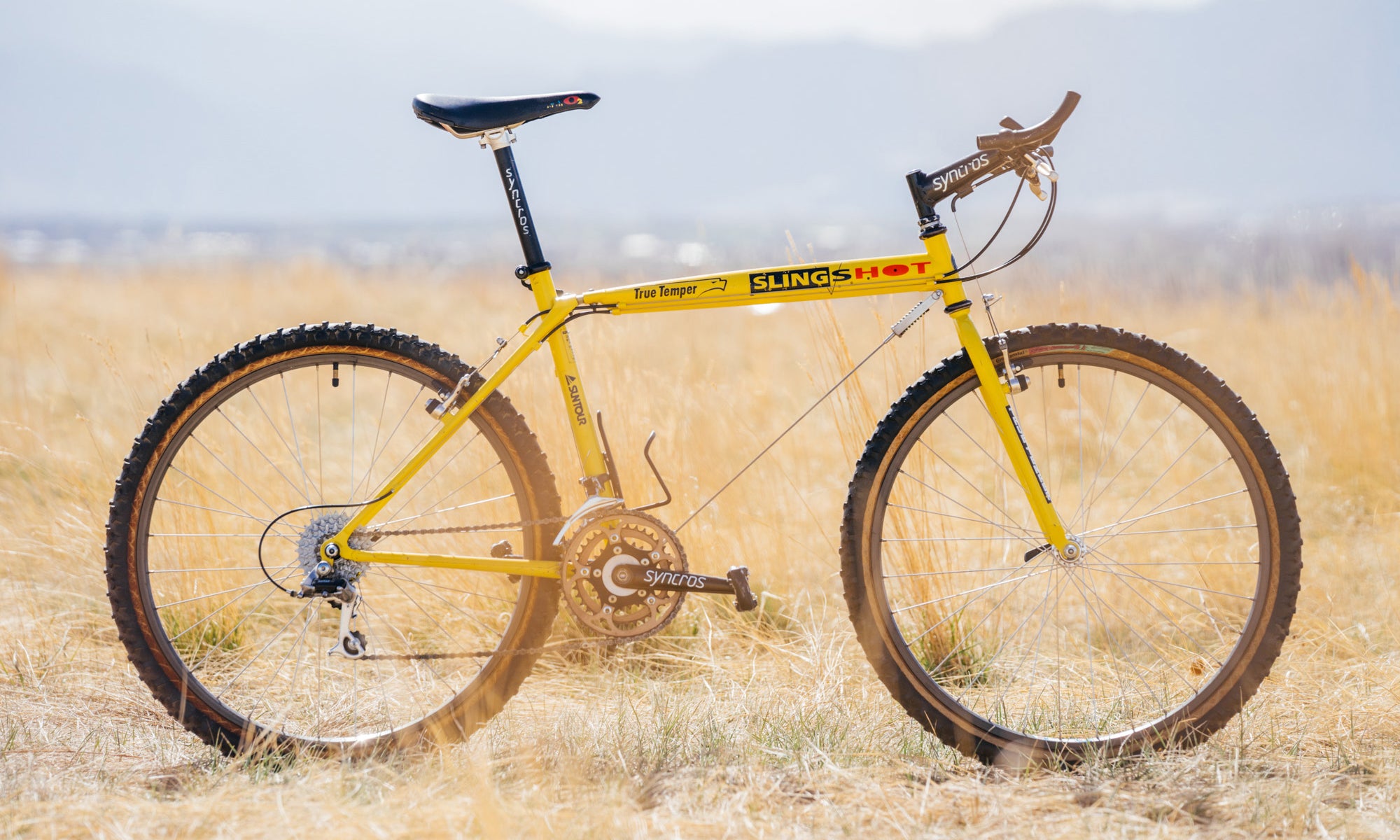A detailed color photograph captures a striking yellow racing bicycle prominently positioned in the foreground amidst a field of long, yellow, dried grass. The bike is angled with its sleek, streamlined shape facing left. Its vibrant yellow frame, emblazoned with the name "SLINGSHOT" and adorned with a stylized eagle and the word "TRUTEMPER," commands attention. A black rectangle on the frame displays the word "Sling" in yellow, with "S" in black and "H-O-T" in red. The slender, agile seat is black and paired with a black pedal system. The handlebars, short and forward-facing, are brown and labeled with "SYNCROS" in white font. 

In the blurred background, a sky of blue-gray hues creates a muted contrast with the bicycle's vivid frame. Indistinct forms suggest either houses or a distant urban scene, with a hint of mountainous terrain in the far distance, adding depth to the composition. This image, devoid of people or animals, captures the solitude and elegance of the bicycle against a backdrop suggestive of an expansive landscape.